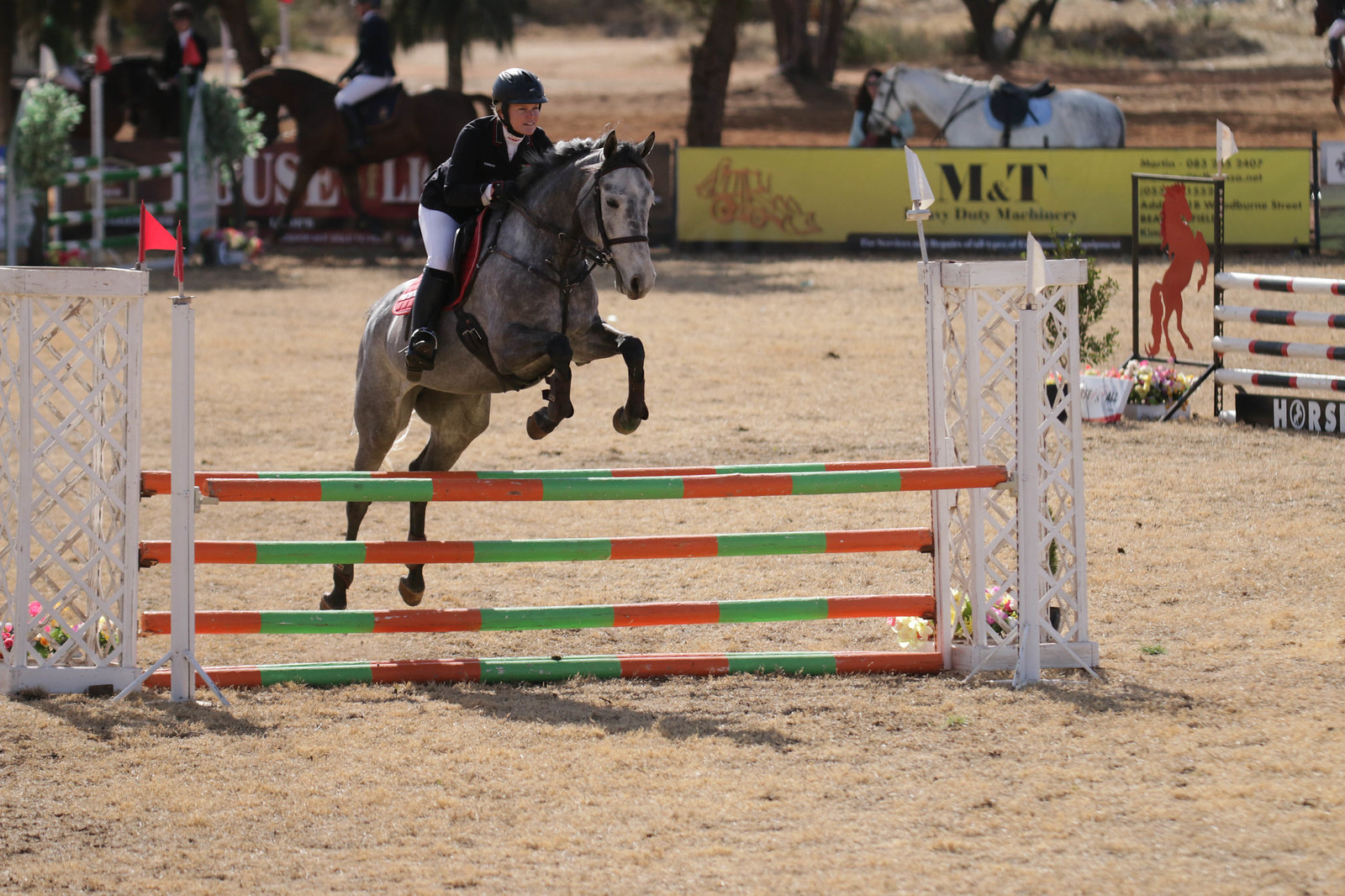In this vivid image capturing the intensity of an equestrian event, a female jockey, distinguished by her black helmet encapsulating her blonde hair, commands attention. She is attired in a sleek black jacket, crisp white leggings, and knee-high black boots, creating a striking contrast against her mount. Her horse, a magnificent grey speckled steed with a blend of white and darker tones, soars gracefully in mid-air over a set of horizontally stacked poles. These obstacles feature a dynamic combination of green and orange bars, integrated between two white, trellis-like structures, forming a challenging leap for the horse. The event takes place on a coarse, medium brown sand arena, surrounded by low-cut, slightly wilted grass. In the backdrop, other participants and horses can be seen, either walking or preparing for their turn, including one horse with its rider standing beside it, perhaps in a moment of camaraderie or strategy. The arena is defined by a chest-high fence, with red flags intermittently placed to indicate the directional flow of the course. This image captures a moment brimming with precision, elegance, and the raw power of the equestrian sport.